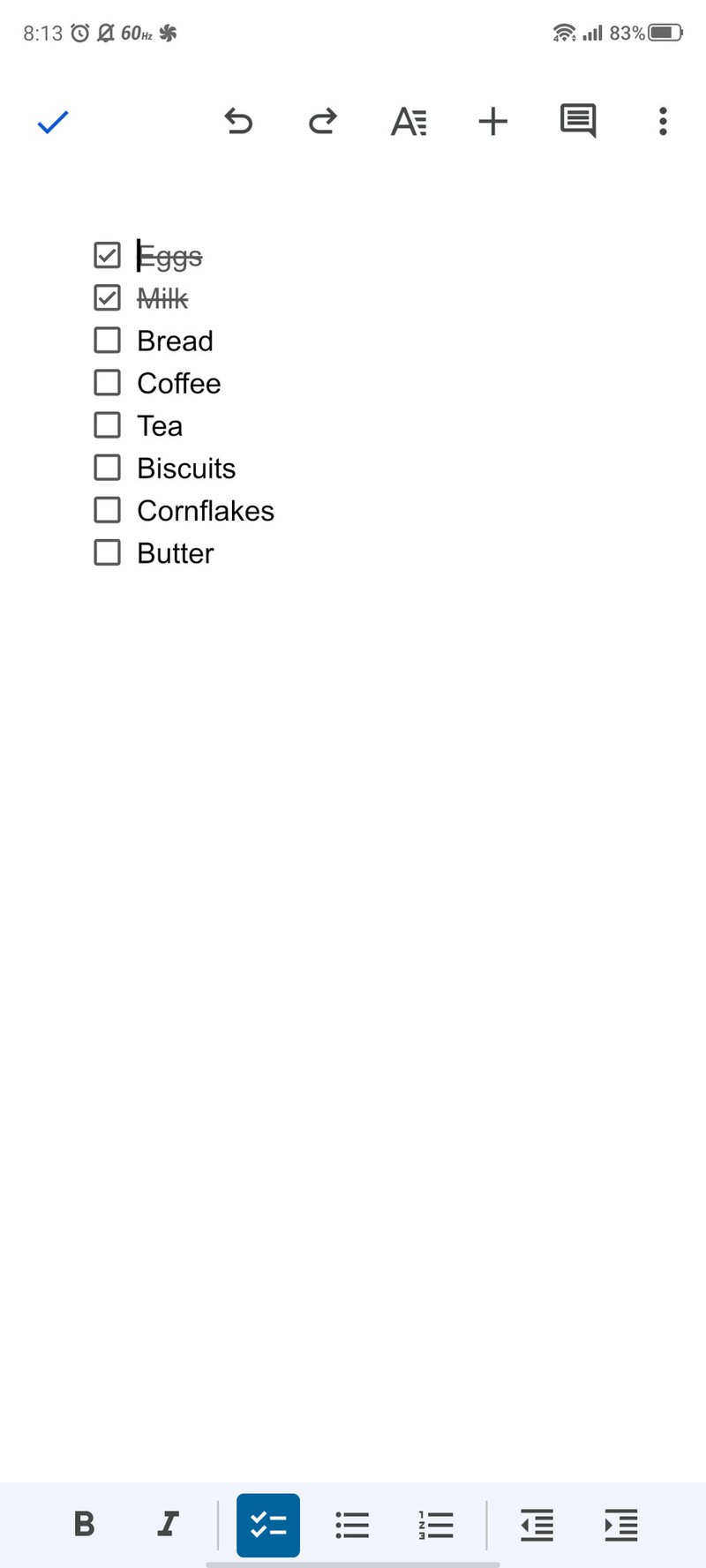This is a detailed descriptive caption for the image:

"A smartphone screenshot showcasing a to-do list application with various icons and features. At the top of the screen, there is a gray header containing text and several icons. The time displayed is 8:13, accompanied by a clock icon, a muted notifications icon, and a '60 HZ' symbol, which indicates the screen refresh rate. Beside these, there is an icon resembling a flower whose function is unclear. On the far right, a strong Wi-Fi signal icon is visible, alongside a battery icon indicating an 83% charge.

Beneath the timestamp, there is a checkmark and an interface comprising a backward arrow, a forward arrow, and an 'A' with horizontal lines to the side, which likely represents text formatting options. Next to these, there is a plus sign, a paper or document icon, and three vertical dots indicating a menu or more options.

The main body of the screenshot lists vertical entries with checkboxes beside them. The first two items, 'eggs' and 'milk,' are crossed out and checked. The remaining items on the list are 'bread,' 'coffee,' 'tea,' 'biscuits,' 'cornflakes,' and 'butter,' all with empty checkboxes beside them.

At the very bottom of the screenshot, there is a toolbar with several icons. These include a 'B' for bold text, an 'I' for italic text, a double checkmark, and three sets of lines or list icons. Additionally, there are right-facing and left-facing arrows accompanied by horizontal lines, though their exact functions are unclear."